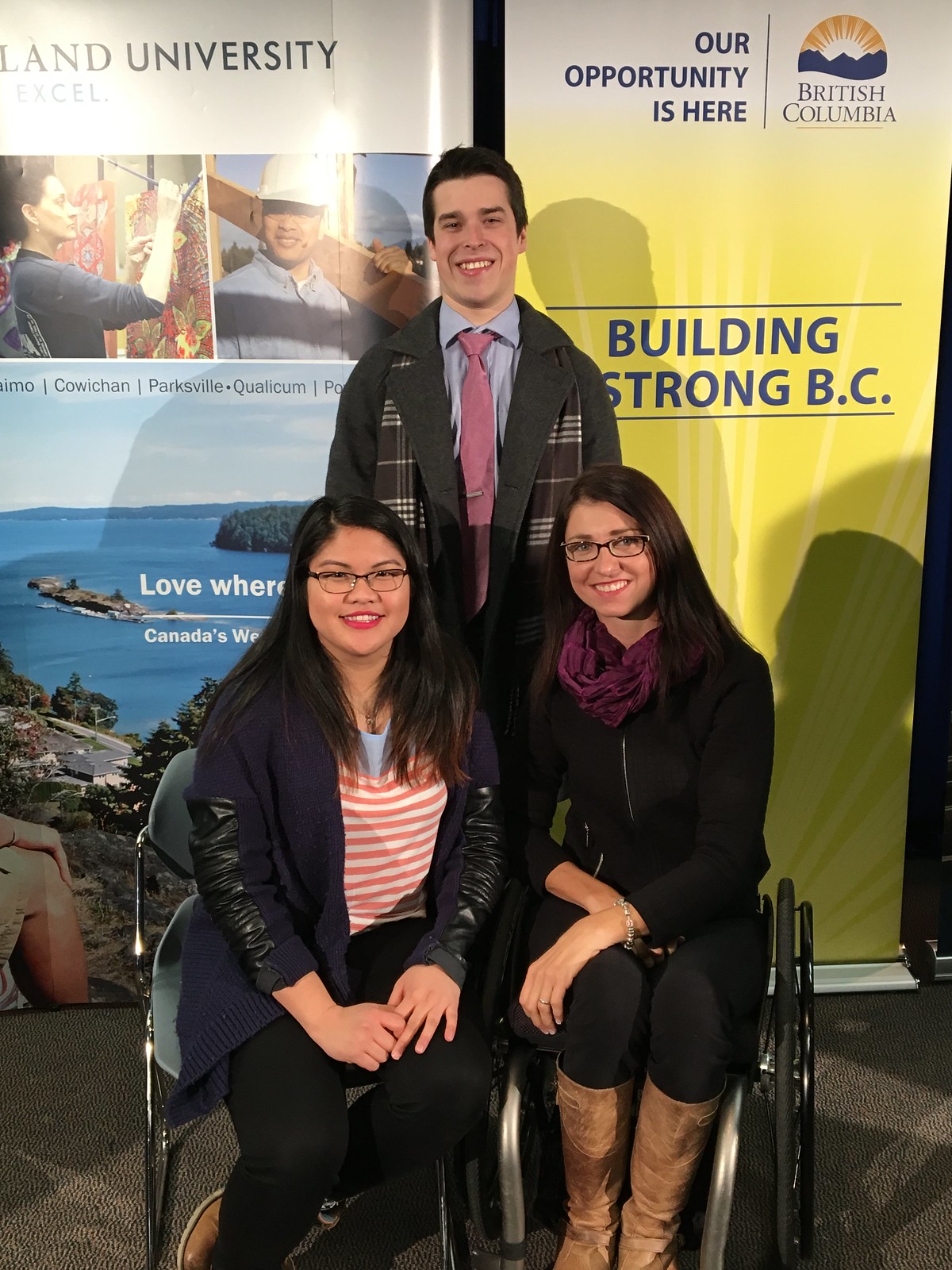The image captures three individuals centered in front of two colorful posters, one of which is for a university and the other promoting British Columbia with the text "Building Strong BC" and the slogan "Our Opportunity is Here" featuring a sun logo. The individuals wear dark attire: the man at the back, smiling, is in a black suit coat with a patterned brown and white plaid scarf and a pink tie, while the two women seated in front of him are both wearing glasses. The woman in the wheelchair, clad in a black shirt, black pants, and brownish gold boots, has a black wheelchair with silver bars. Next to her, the other woman, of Asian descent, is dressed in a deep purple wool jacket and black pants. The photograph showcases them posing at an event celebrating British Columbia, with a backdrop of diverse, colorful signs.